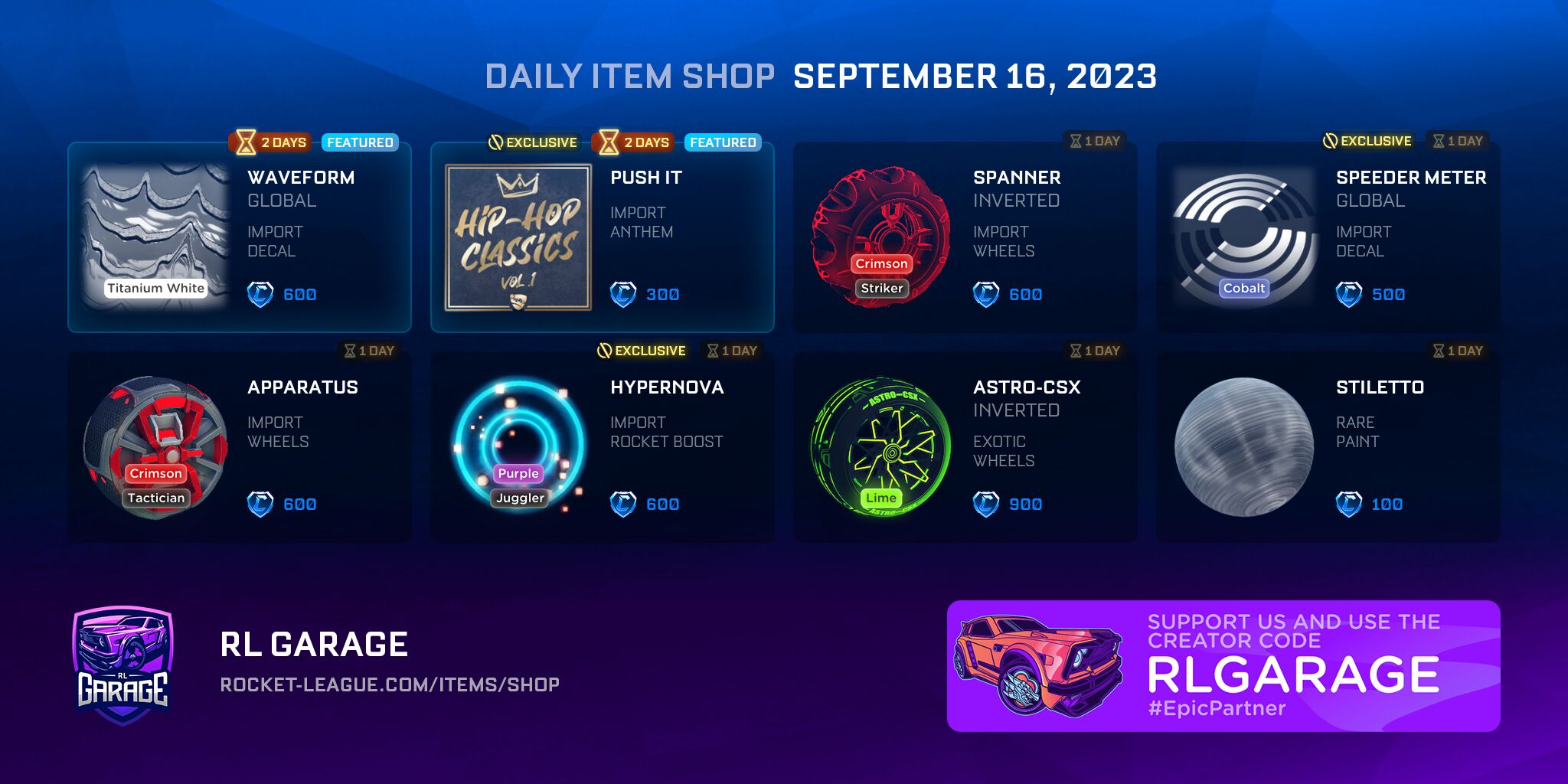In this detailed image of the Rocket League Garage interface, the top portion features a blue background in varying shades of darker blue. In bold text, it reads "Daily Item Shop, September 16th, 2023." An RL Garage icon is prominently displayed on the left, accompanied by the website link rocket-league.com/item/shop. Additionally, there's a logo promoting support for the creators, encouraging users to use the creator code RL Garage, marked with a hashtag Epic Partner.

The primary section of the image showcases various items available in the shop. Among them are two special featured items: a Titanium White 'Wave Form' Global Import decal priced at 600 Rocket League credits and 'Push It,' an Import Album from Hip Hop Classics Volume 1, available for 300 credits.

Additional items include:
- 'Spanner Inverted' Import Wheels in Crimson Striker for 600 credits.
- 'Speed Meter' Global Import decal in Cobalt for 500 credits.
- 'Apparatus' Import Wheels in Crimson Red Tactical for 600 credits.
- An exclusive 'Hypernova' Import Rocket Boost in Purple Juggler for 300 credits, which tracks certain in-game skills.
- 'Astro CSX' Exotic Wheels for 900 credits.
- 'Stiletto' Rare Paint for 100 credits.

This comprehensive display neatly organizes the available items, complete with detailed descriptions and prices, catering to the needs of Rocket League enthusiasts.